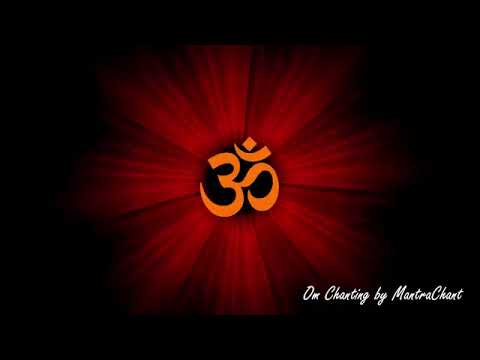The image, which appears to be the cover of a book or a music CD/album, is primarily black with a central design featuring a dark red, muted radiating color that suggests emanation from the middle outwards. At the core of this design is a symbol resembling the number three, with additional elements such as a half-circle, a horizontal line above it, and a small circle situated at the top. This central symbol gives off a glowing effect, intensified by the red color accents that fade into the surrounding black space. In the lower right corner, there is white cursive text that reads, "Ohm Chanting by Mantra Chant," signifying the likely spiritual or meditative theme of the content. The overall design is simplistic yet striking, focusing attention on the symbolic middle and the elegant script at the bottom.